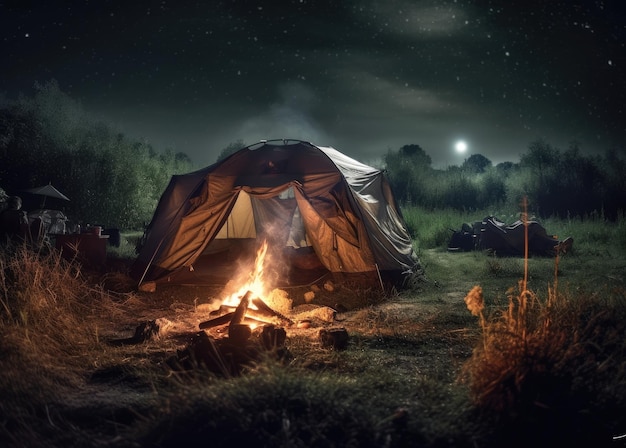This detailed photograph, possibly computer-generated due to its hyper-realistic quality, captures a nighttime camping scene set in a lush, green wilderness, likely during spring or summer. Dominating the foreground is a spacious, white tent, open at the front and illuminated warmly by a blazing campfire. The fire is encircled by logs, indicating a communal sitting area. To the left of the tent, a small umbrella and table suggest a designated dining or picnic spot, while to the right, a pile of wood is seen, prepared for sustaining the fire. Trees, wild grass, and brush frame the scene, contributing to the natural and untamed ambiance. No people are visibly present within the image, though there is a faint, distorted impression that might be someone lying down inside the tent. The background features a dark, star-studded sky with patches of clouds, and a large, low-hanging moon, intensifying the nightscape’s moody atmosphere. Despite some elements hinting at possible digital manipulation, the overall scene conveys an authentic and serene camping experience.